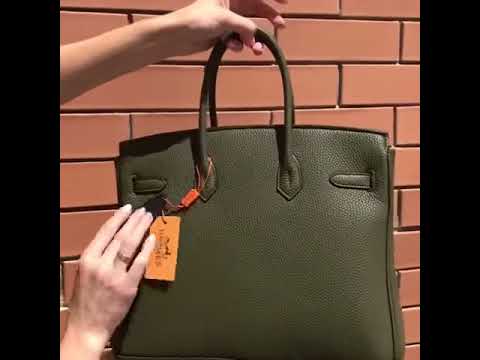In the image, a woman's hands are prominently displayed, showcasing a designer bag against a backdrop of what appears to be a faux brick wall with thin, vertical black bars. The bag, which is a dark beige or olive-green leather, is presented in the center of the frame. She holds the bag's handle with her left hand, gripping the top with her thumb, ring, and pinky fingers. Her right hand, adorned with a silver ring on her ring finger, steadies a light brown, possibly cardboard tag with a string, which hangs from the orange strap at the front handle. The scene suggests the bag is for sale, highlighting its details and tags as if in a product display or still from a promotional video.